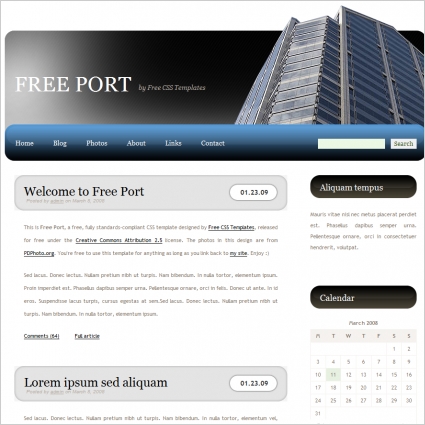This screenshot captures the detailed layout of a website template called "Freeport." At the top, a sample image of a skyscraper, extending beyond a gradiated black and white banner, is prominently displayed. The banner features the text "FREEPORT" in large, uppercase white letters, accompanied by "Buy Free CSS Templates" in smaller white fonts, indicating the template's free status. Below the banner lies a navigation bar with a gradient transitioning from light blue to black, containing links to Home, Blog, Photos, About, Links, and Contact pages, and a search bar situated on the right.

In the content area below, the template showcases various elements standard to a blog or website. To the left is a gray block with a welcoming headline, "Welcome to Freeport," followed by a date (01.23.09) and placeholder text ("Lorem Ipsum Sed Aquilum"). Another column beneath the search bar features additional placeholder text, suggesting areas for a website bio, sample text, or descriptions, all set against a white background with dark gray writing and black fonts for section headers. A calendar dated March 2008 is also present, demonstrating the sample structure and editable elements of the template. Overall, this Freeport template provides a comprehensive and editable foundation for anyone looking to kickstart the creation of a website or blog.